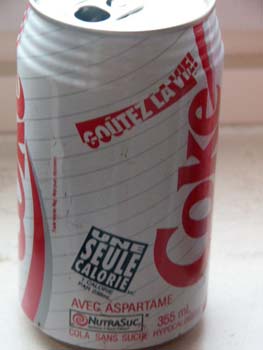The image depicts a vintage, foreign Diet Coke can that has already been opened, sitting on a wooden table with light coming from behind it. The can, featuring a white background with red designs, showcases the classic Coca-Cola logo vertically written and includes a French slogan at the top. The slogan reads "Que des la vie" and "Une Seule Calorie," emphasizing its low-calorie content with the use of aspartame as a sweetener. The can also notes its volume as 355 milliliters, consistent with the metric system. An interesting feature of this can is its slightly rippled and terraced top edge, which differs from typical smooth Coca-Cola cans. The design includes fine silver stripes encircling the can.